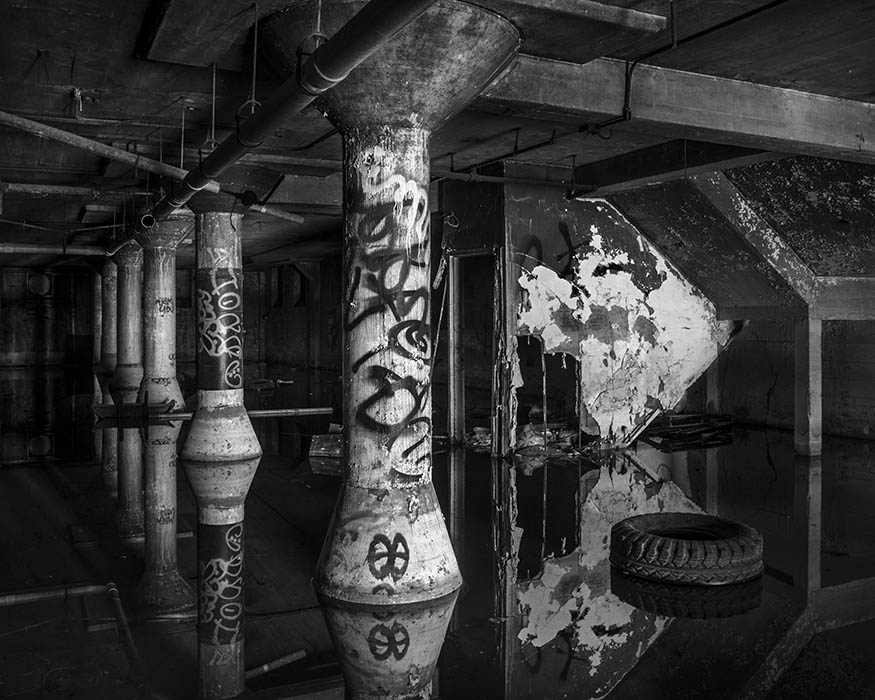The image is a black and white photograph depicting a flooded underground tunnel or basement-like area. The floor is covered in water, creating a reflective surface that clearly mirrors a tire lying on the right side, nearby white walls, and scattered rubble in the background. The central and far background is lined with a series of concrete pillars, some cylindrical and others rectangular, stretching into the distance. Several of these pillars, particularly the central ones, bear vibrant graffiti art despite the grayscale palette of the photo. Broken pipes are visible both on the floor and ceiling, hinting at structural decay and neglect. The ceiling is visible and contributes to the overall desolate ambiance, accentuated by the presence of trash and debris scattered throughout the scene. The overall composition suggests an abandoned, deteriorating infrastructure, possibly part of an old parking deck or storage facility.